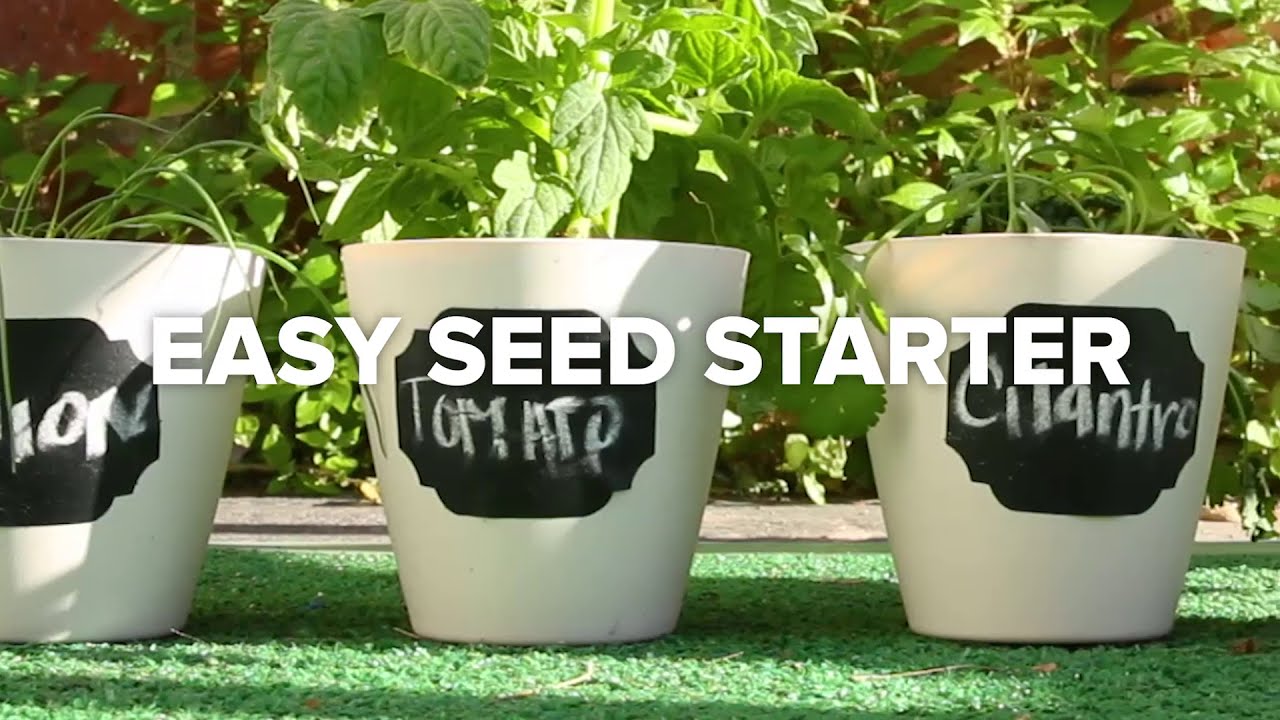The image features three white ceramic pots neatly arranged in a row, each adorned with a black chalk label displaying handwritten text in white. From left to right, the labels identify the plants as Onion, Tomato, and Cilantro, though the Onion label is partially obscured. Each pot contains its respective plant, with green shoots emerging prominently. The scene is set against an artificial grass surface, transitioning to a stone-like texture further back. In the background, an assortment of additional vegetation and possibly a red brick wall are visible, casting shadows indicative of bright sunlight. Bold white block letters across the middle of the image proclaim "Easy Seed Starter."